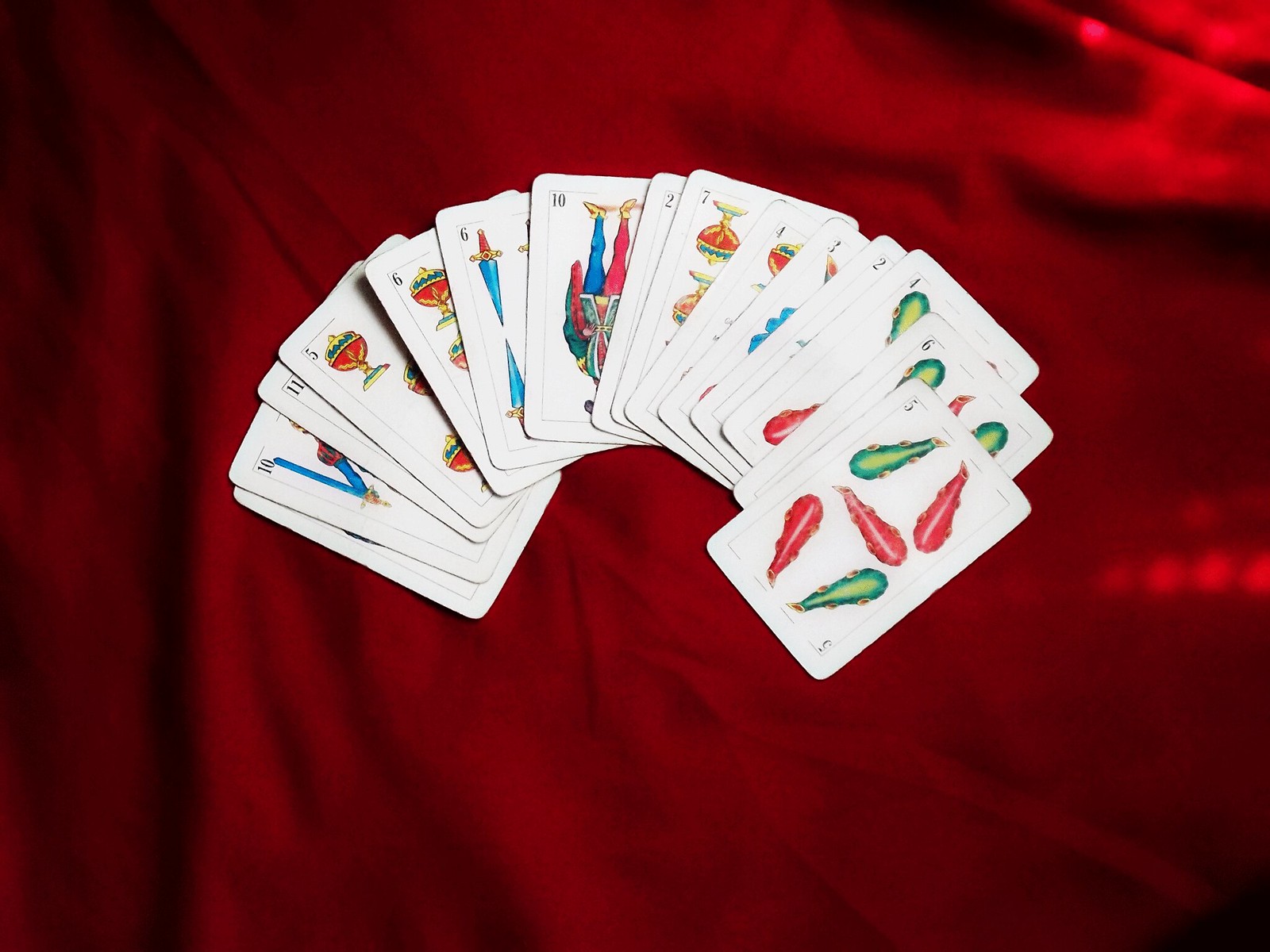The image features a rectangular area with a vibrant red background, upon which a deck of cards is meticulously laid out in a fan shape. To the far right of the deck, one card is prominently faced up, displaying a charming illustration of three orange fish and two green fish. This card draws immediate attention, standing out against the array of largely face-down cards.

Approximately eight cards away from the rightmost card, another card's details become discernible. This card is an upside-down Jack or King, distinctive for its attire - one blue pant leg and one red pant leg, paired with an ornate jacket. Due to its orientation, the intricacies of the head design remain unclear.

To the left of this card lies another card marked with the number six, adorned with blue swords. Adjacent to it, another six appears, this one embellished with intricately designed canisters. Continuing left, the next card features the number three and bears a similar decorative theme as the six.

Further to the left are partial views of two more cards: one with the number eleven and another with the number ten. An arm holding a sword is visible on one of these partially concealed cards. Lastly, there is one card at the very edge of the fan where no details are discernible, leaving it a mystery.

Overall, the arrangement of the cards and the vivid colors create a visually engaging composition.